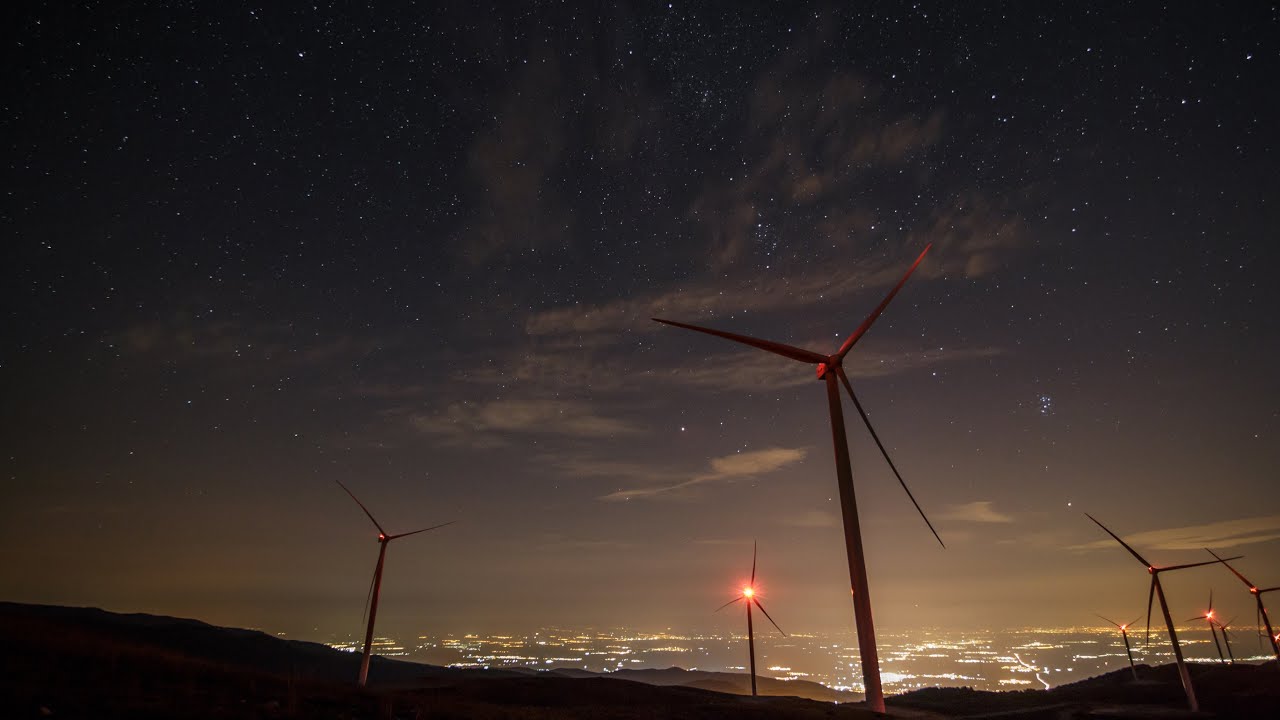This nighttime photograph captures a serene, almost mystical scene as the sky transitions from twilight to night. A faint golden glow clings to the horizon where the land meets the evening sky, hinting at the recently departed sun. Above, the darkening sky begins to twinkle with stars, their faint white flecks piercing the growing darkness. The star-speckled firmament shares space with clusters of scattered clouds, adding texture to the night.

The photograph's foreground features several wind turbines with red lights, standing tall on a hilly terrain overlooking a sprawling metropolis. These turbines, marked with bright red lights to signal low-flying aircraft, create a stark contrast against the sky. Their silhouette forms, often in a Y shape, are illuminated subtly by the red glows.

In the distance, the city lights sparkle and shine, showcasing a bustling, vibrant metropolis. The cityscape, with its myriad lights, lends an air of constant activity against the calm of the starry sky and the quiet sentinels on the hills. This horizontally framed, rectangular photograph encapsulates the beautiful intersection of nature and human ingenuity in a single, captivating night scene.